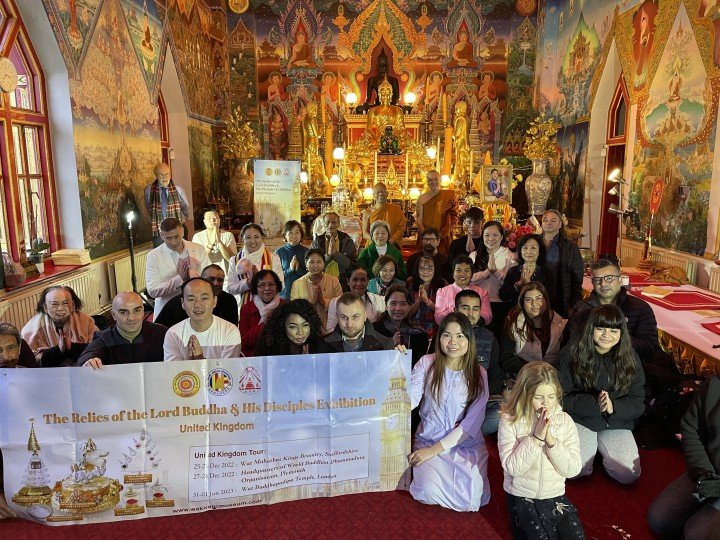This photograph captures an indoor scene within a small, ornate room of a church or cathedral, taken during the daytime. The rectangular image, approximately six inches wide and four inches high, reveals the left, back, and right walls of the room, adeptly showcasing the intricate decorations. The floor is covered with a thick red carpet, adding warmth to the scene.

Dominating the center of the room is a gold statue of Buddha, surrounded by intricate paintings of religious icons and various colorful details that grace the walls. The window on the left allows sunlight to stream in, enhancing the room’s serene ambiance.

Kneeling on the ground, facing the camera, is a diverse group of people, most with their hands together in prayer. While many appear to be of Asian descent, there are a mix of ethnicities present. On the left, several individuals hold a large, white, rectangular banner with gold print. The banner reads, "The Relics of the Lord Buddha and His Disciples Exhibition, United Kingdom," and includes details about the United Kingdom tour, dated December 2022. Ornate jeweled statues are displayed to the banner’s side, adding to the richness of the scene.

In addition to the Buddha statue, two monks, dressed in traditional orange robes, are positioned near the altar, further emphasizing the room's sacred and ritualistic atmosphere. The room's elaborate decor features predominantly yellow, gold, and white tones, interspersed with splashes of purple, blue, green, and other colors, contributing to the photograph's vivid and detailed portrayal of a spiritual gathering.